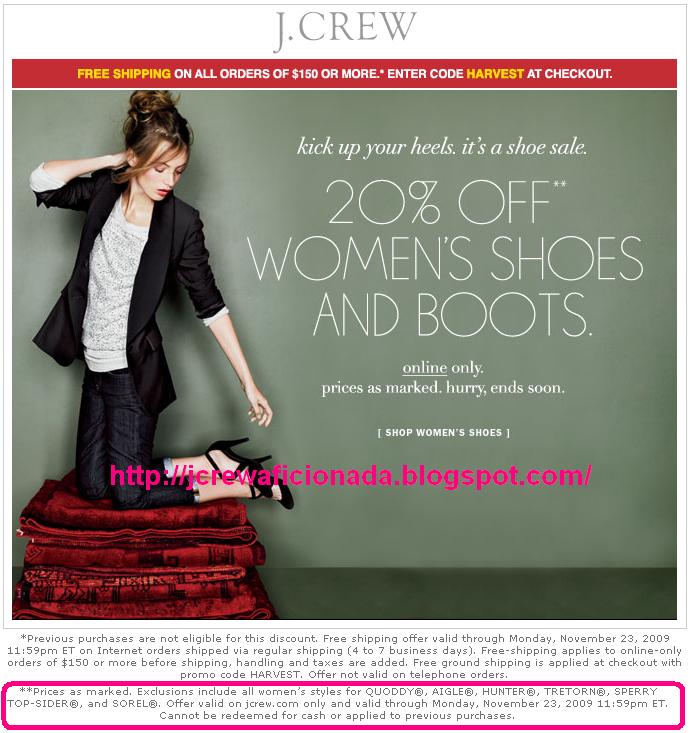Here's a detailed and cleaned-up caption for the image:

---

"This screenshot from the J.Crew website features a sophisticated and elegant design. At the top, the J.Crew logo is prominently displayed in a stately gray font. Directly below, a vibrant red banner announces, 'Free shipping on all orders $150 or more,' with an asterisk for further details. The phrase 'Free shipping' and the promotional code 'HARVEST' are highlighted in gold, while the rest of the text is in white. 

Beneath this banner, a promotional image captures attention. It depicts a woman kneeling on a pile of red linens, which vary in patterns and textures. She is dressed in stylish black pants and a matching black jacket over a white shirt. Her chestnut hair is styled up in a bun, with a few loose bangs framing her face. Her eyes are closed, giving a serene expression as she looks down to her right. Her pale complexion is complemented by a subtle touch of lipstick.

To the right of the image, bold text reads, 'Kick up your heels, it’s a shoe sale. 20% off women’s boots and shoes. Online only. Prices marked. Hurry, ends soon. Shop women’s shoes.' A bright pink watermark indicates that the image is shared from jcrewaficionada.blogspot.com. 

At the bottom of the screenshot, two disclaimers provide detailed information regarding the free shipping offer and the 20% discount on women’s footwear. The disclaimer associated with the shipping banner is marked with an asterisk, while the one related to the footwear sale is outlined in pink text for emphasis."

---